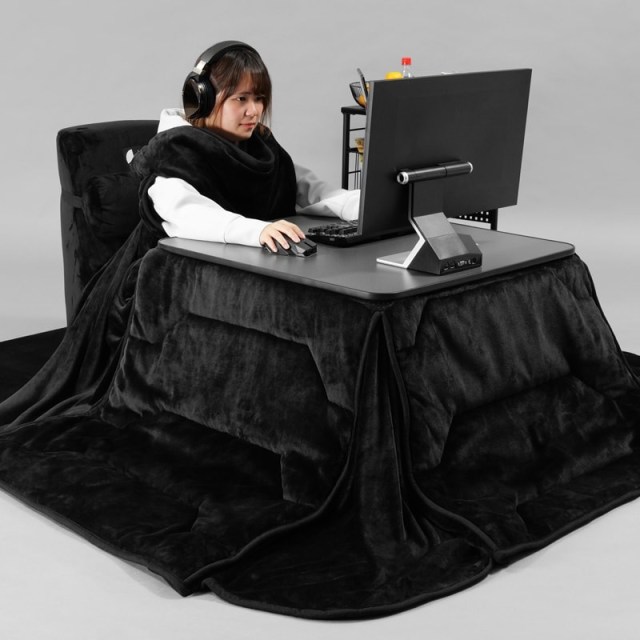The image is a carefully crafted Photoshop-style photograph displaying a scene where a woman, or possibly a girl, sits at a desk, presenting an illusion that visually merges elements of a workspace and a bedroom setup. She is engaged with her computer, wearing headphones, with her right hand on a mouse and her left hand manipulating a keyboard. The desk appears to be transformed into something reminiscent of a miniature bed through the creative use of a velvety black fabric. This thick, fleece-like covering drapes over the desk and extends down to the floor around all sides, creating an impression comparable to a bedspread. The same black fabric cascades behind the woman and is also draped over portions of her body, contributing to the surreal and cozy atmosphere. The desktop itself remains partially visible, especially around the mouse and keyboard areas, maintaining a light gray contrast against the dark cloth. The desk chair takes on the appearance of a fuzzy headboard, suggesting the woman is comfortably nested within a bed while working. Despite the realistic appearance of the subject, the photograph lacks typical functional details like visible power cables, highlighting its nature as a likely product display for the luxurious blanket enveloping the scene.